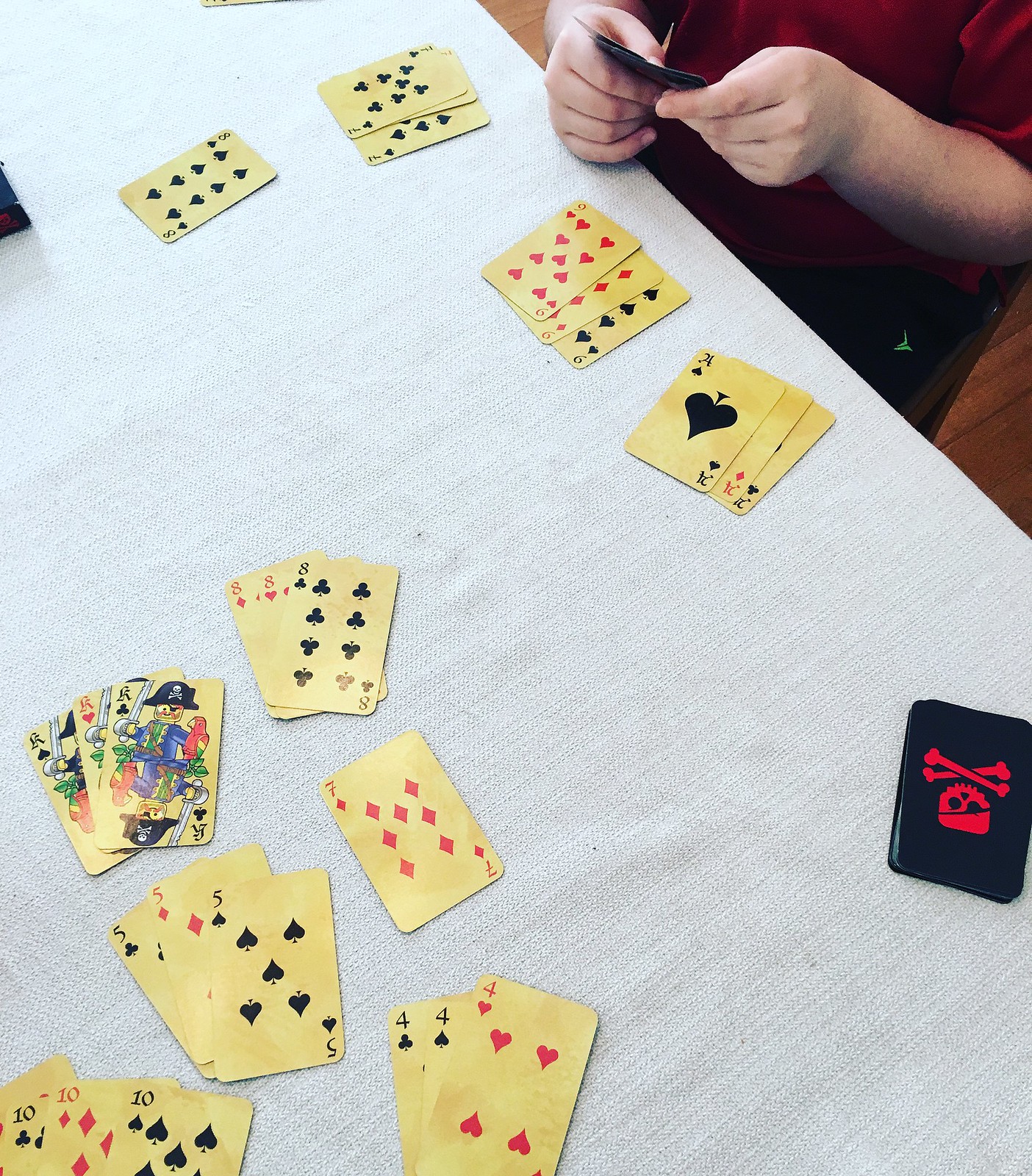An overhead shot captures an individual engrossed in a card game, their bare arms and wrist visible as they scrutinize their hand. The scene is set on a white tablecloth, emphasizing the contrast with the worn, beige cards scattered across the surface. The player appears to be holding six or seven cards, among them three matching cards and potentially an ace. Situated in the center of the table is a distinctive deck of cards, marked by a black skull and crossbones emblem. These cards exude an antique charm, showing signs of heavy use. The face cards intrigue with their pirate-themed illustrations, depicting queens, kings, and jesters in a swashbuckling style.